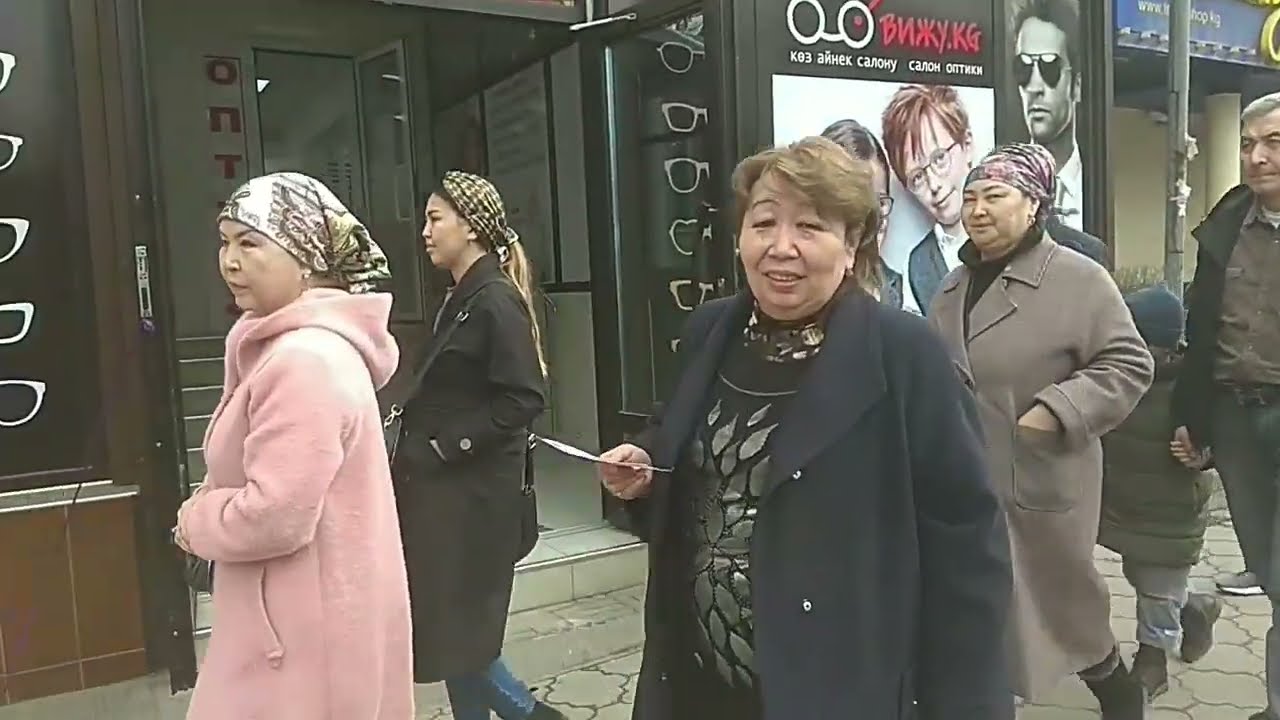In this daytime urban scene, an older Asian woman, perhaps in her 60s, stands out as the focal point. She wears a large navy blue peacoat over a black shirt adorned with green accents, and her short light brown hair frames her face as she looks directly at the camera. Surrounding her, a diverse group of pedestrians, predominantly older women except for one man holding a child's hand, walk along a concrete walkway. This busy street, lined with various storefronts adorned with advertisements (including one for glasses written in Russian), captures a moment of everyday life in what appears to be a bustling city center. The image features a palette of black, white, brown, gray, pink, dark blue, silver, purple, and yellow, adding vibrancy to the scene.